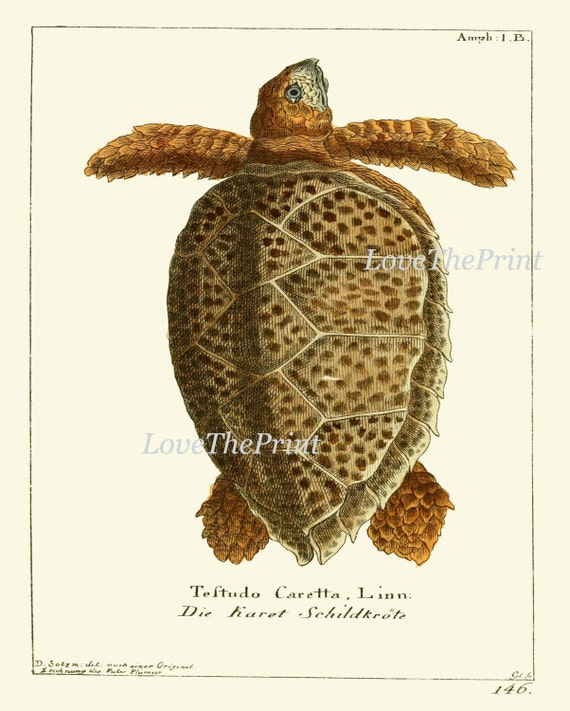This detailed illustration appears to be a page (numbered 146) from a book, featuring an artistic depiction of a turtle. The turtle is rendered with brown limbs and a shell that is predominantly beige with brown spots. Uncharacteristically, its long arms seem to emerge from its neck, lending it an unnatural appearance. The turtle boasts distinctive blue eyes and a beige-toned mouth. The image includes the text "Love the print" twice, positioned at the top of its shell and again at the bottom. Below the turtle, in different languages—one of which resembles German—the text "Teptudo Coretta Lin" or similar variations can be seen. The turtle is encased in a black outline, enhancing its illustrated, rather than photographic, nature.